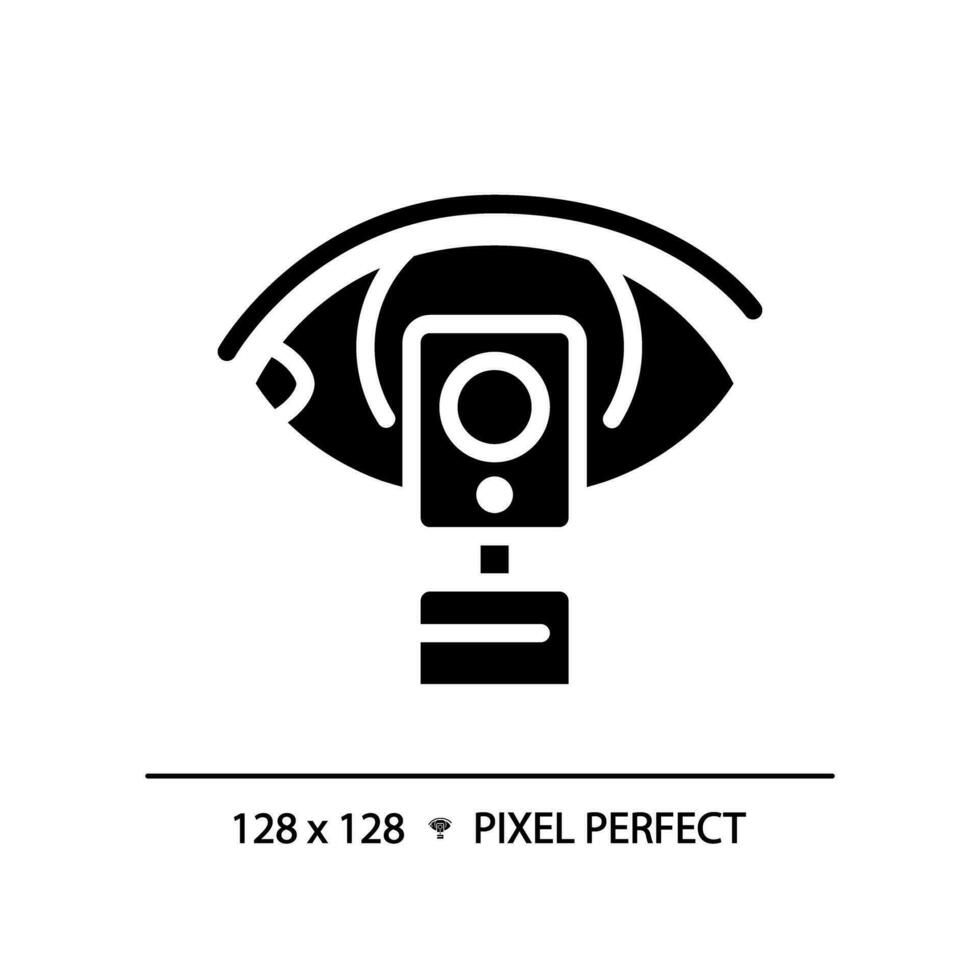This image showcases a detailed artistic render of a corporate logo against a completely white background. At the bottom, the text "128x128 pixel perfect" is written in a clean black font. A thin black line, situated about an inch above this text, separates the labeling from the main icon. The logo itself is a monochromatic depiction of an eye integrated with a camera, all elements rendered in black and white.

The core of the logo features a black almond-shaped eye with two white semicircles highlighting the left and right sides of the almond, creating a striking visual representation of the eye. Inside the almond shape, there is a smaller black circle that represents the pupil, embedded within a larger white circle occupying the top two-thirds of a vertical black rectangle. This vertical rectangle also includes another smaller white circle near its bottom. Directly beneath this structure lies a small black square, and below that is a more sizable black rectangle with a white line segment cut through it, giving the impression of part of a camera’s body.

Floating above the eye is a black, slightly curved line reminiscent of an eyebrow, enhancing the visual symbolism of the eye gazing through the camera lens. The eye's iconic representation within the camera design gives the logo an inventive twist, merging the themes of vision and technology seamlessly.